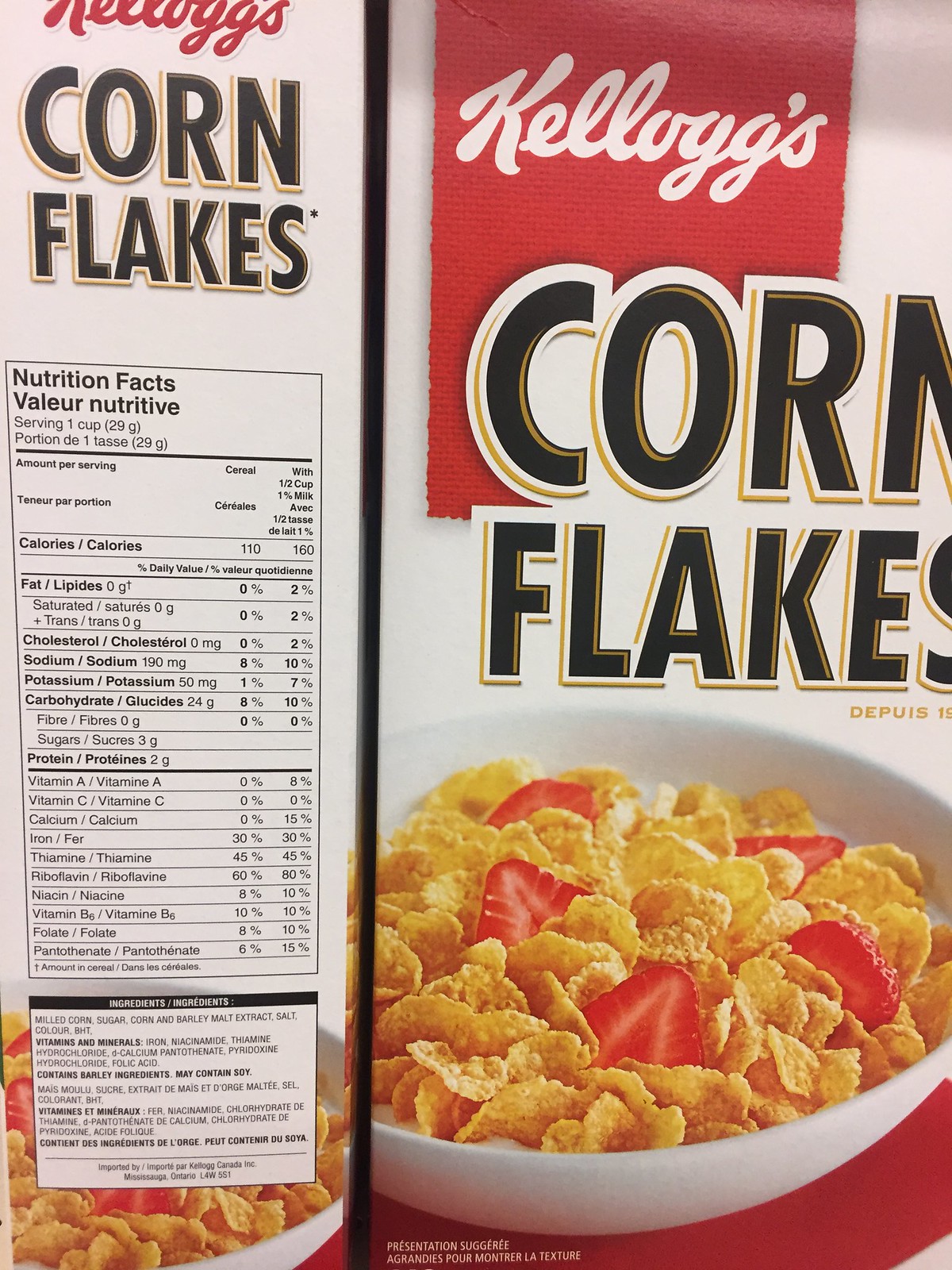This image showcases a flattened Kellogg's Corn Flakes cereal box, presenting both the front and side panels clearly. The main front panel features a predominantly white background with a striking red flag in the top-left corner, emblazoned with the "Kellogg's" logo in white lettering. Below, the product name "Corn Flakes" is prominently displayed in black letters, highlighted by gold and white accents. Dominating the front panel is a large, inviting bowl filled with golden Corn Flakes, milk, and chopped strawberries, resting on a vibrant red cloth. On the side panel to the left, the "Kellogg's" branding continues in red, along with "Corn Flakes" written in black. Additionally, this side panel provides the nutritional information for the cereal.